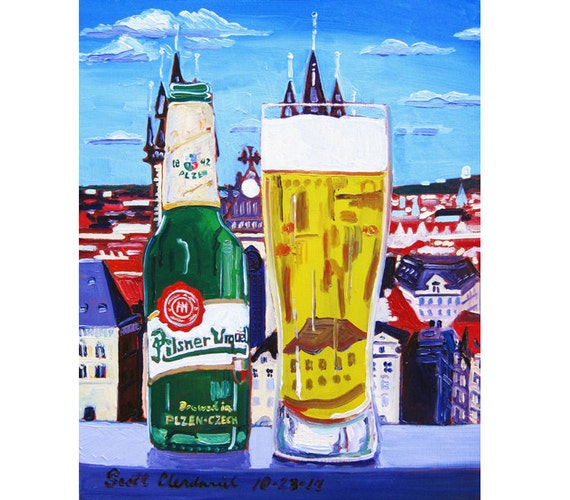This detailed watercolor portrait captures a green glass bottle of Pilsner beer on the left, featuring a distinctive white label and red branding, next to a tall beer mug filled with clear yellow liquid and topped with a generous foamy head. Both beverages rest on a white railing with a painted blue bottom, resembling a ledge or porch. Behind the drinks, a cityscape unfolds, characterized by blue- and red-roofed white buildings and prominent church steeples, suggesting a European town. The scene is set under a bright blue sky dotted with clouds. At the lower part of the painting, the artist's signature and the date 10-23-14 are visible.